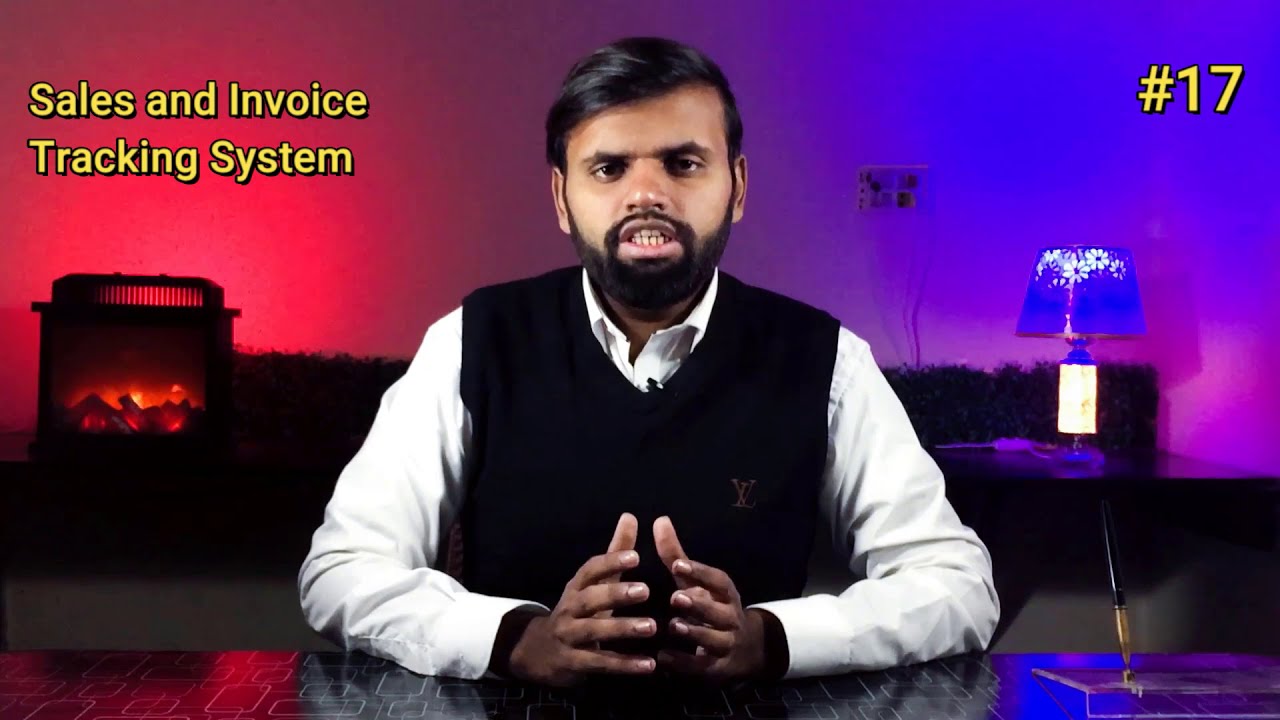In this photorealistic image, a South Asian man is seated centrally at a table, facing the camera. The man, who has short black hair, a black beard, and is wearing a white dress shirt with a black vest, appears to be speaking, his mouth open with his lips parted but teeth together. His hands are resting on the table, which is black with rectangular silver-outlined patterns. He is illuminated by contrasting lighting—the left side bathed in a reddish glow from a fake fireplace with simulated flames, and the right side highlighted by a blue light from a desk lamp with a blue shade adorned with a white flower pattern. The background suggests an indoor room setting. On the upper left of the image, yellow text reads "Sales and Invoice Tracking System," while on the upper right, the text "£17" is prominently displayed in yellow font. A device with visible wires is also noticeable on the wall closer to the lamp.